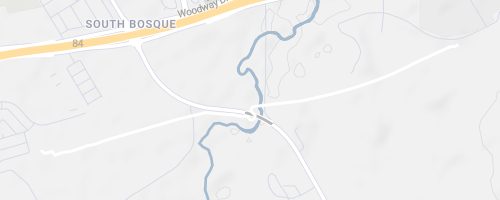The image depicts a detailed, small section of a horizontal rectangular map. The background is predominantly light gray, featuring an orange-colored road labeled with the number 84 that moves diagonally from the top left to the top center of the image. This road is prominently curved. Intersecting this orange road is a faded white road that enters from the top left, veers downwards and to the right, then curves upwards and extends to the top right before stopping just shy of the image's edge. At the intersection of these two roads, “South Bosque” is visibly marked. To the right of this intersection, in smaller text, are the words "Woodway."

A curvy blue line, perhaps representing a river or creek, stretches from the top center, slithers to the left, curls back to the right, and plummets straight down the image before shifting leftward and eventually exiting near the bottom left. Another white road emerges from the bottom left corner, arches upwards and to the right, intersects beneath the other white road, and then continues downward, exiting near the bottom right of the map section. The map also contains other faint gray lines and elements, but they are not distinctly identifiable. The overall style of the map is a color illustration, emphasizing the roads and water features in vivid hues against the subdued gray background.